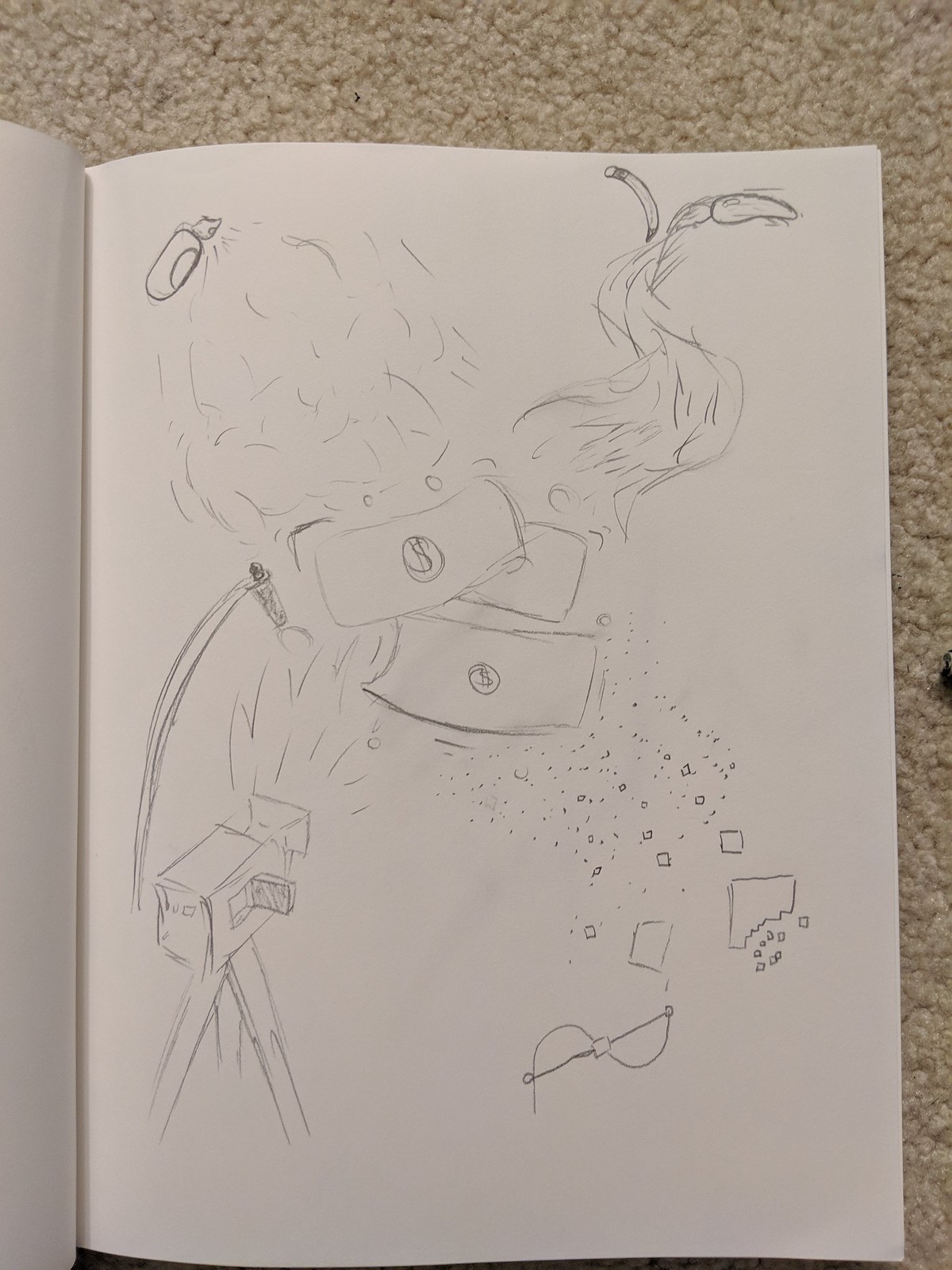In the background of the photo, a beige carpet is visible at the top and right sides. The centerpiece is a child’s pencil drawing on plain white paper from a sketchbook, which is open to reveal another blank page beside it. The drawing features a camera on a tripod positioned in the lower left corner, resembling equipment used for filming movies or TV shows. The camera is pointed upward, and nearby are dollar bills with circled dollar signs, depicted in a burning state with flames and smoke ascending. Above this, there's a smoke detector going off in the upper left corner. Scattered around are various details, including debris in the bottom right corner, possibly broken glass or abstract confetti-like elements, and additional unidentifiable objects such as a bent pencil and cylindrical shapes on the right. Despite the lack of color, the sketch is intricate, capturing dynamic motion and chaotic elements, hinting at a storyboard-like narrative.